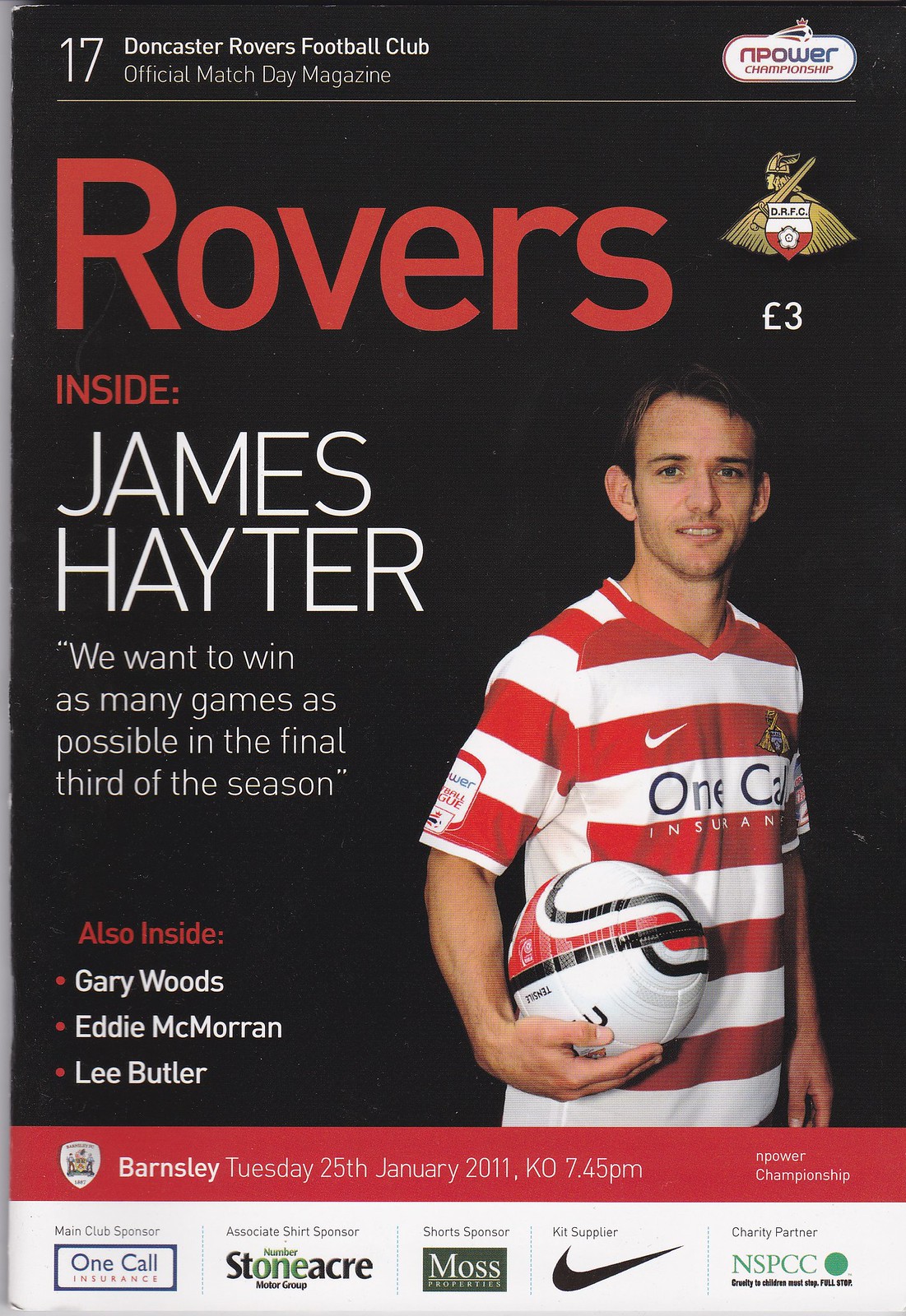Presenting the official match day magazine for the Doncaster Rovers Football Club, Issue 17, dated January 25th, 2011. The cover features a young man with short brown hair and fair skin, awkwardly smiling at the camera while holding a white and black soccer ball under his right arm, and dressed in a red and white striped shirt branded with the OneCall Insurance logo and a Nike swoosh. Headlining the black background in bold white letters is "17 Doncaster Rovers Football Club Official Match Day Magazine," with a large red "Rovers" beneath it. Featured prominently to the left of the player, James Hayter, is his motivational quote: “We want to win as many games as possible in the final third of the season.” Additional features include profiles of Gary Woods, Eddie McCarron, and Lee Butler. The bottom of the cover details the match particulars in white text over a red bar: "Barnsley, Tuesday, January 25th, 2011, KO 7.45 PM, Empower Championship." Sponsors such as OneCall Insurance, Stoneacre Motor Group, Moss Properties, Nike, and the charity partner NSPCC are identified, alongside a distinctive logo of a Viking holding a sword, draped with a red and white shield. Priced at three pounds, this edition captures the spirit and anticipation of the upcoming game in the Empower Championship.